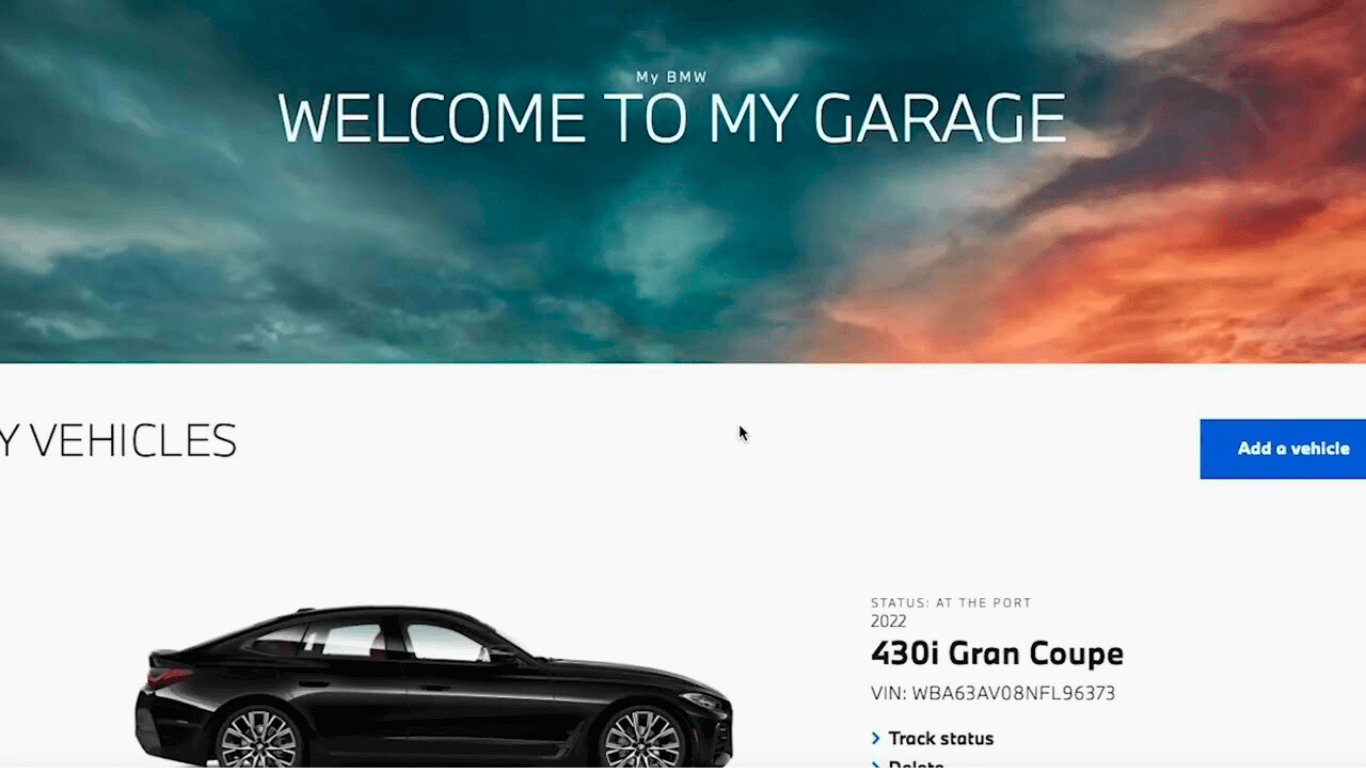The screenshot shows a web page viewed on a laptop or desktop computer in landscape mode. The top of the page features a large banner with a dark, moody cloudscape in shades of blue and white, merging into pink and purple hues on the right side, resembling a sunset. In the upper third of the banner, the text "MYBMW" appears in small white letters, and directly below, in much larger all-capital letters, it reads "WELCOME TO MY GARAGE."

On the left side of the page, a section labeled "MY VEHICLES" is visible. On the right side, there is a button that says "ADD A VEHICLE." The web page appears to be designed for BMW owners to manage multiple vehicles. The user has added one car to their "MY VEHICLES" section, which is listed as "STATUS AT THE PORT," indicating it has not yet been delivered. This vehicle is a 2022 BMW 430i Gran Coupe. The VIN number is displayed in small letters below this information, along with a "TRACK STATUS" option.

The image of the car is partially visible, with the wheels slightly cut off at the bottom. The hubcaps can be seen, and the vehicle is identified as a black, two-door coupe.